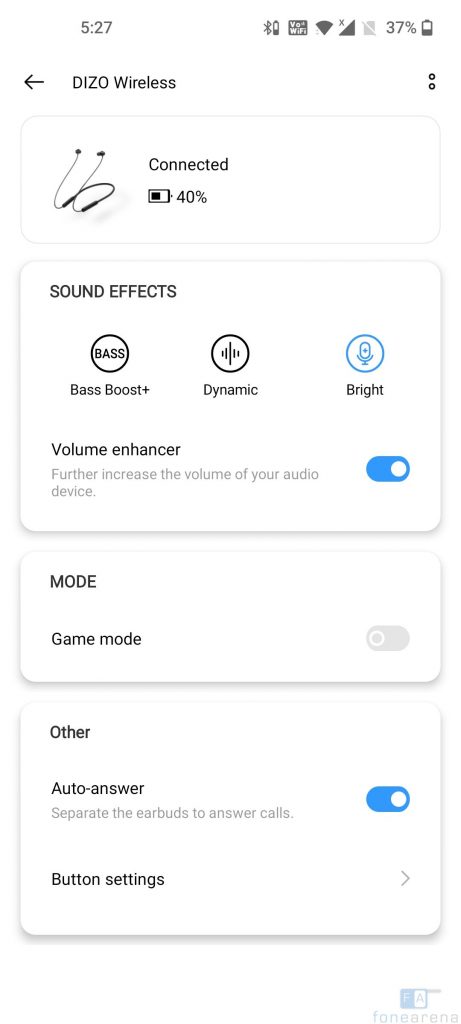On this page, the top section displays the time as "5:27" along with a battery icon indicating "37%" and a Wi-Fi icon showing connectivity status. Below this, there is a navigation bar featuring a left arrow and the label "Diesel Wireless." The main interface features an image of wireless headphones, marked as "Connected 40%." Beneath this image, several audio settings are listed: "Sound Effects" offers options such as "Fast Boost Plus," "Dynamic," and "Bright" (with "Bright" highlighted in blue). The "Volume Enhancer" is switched on, with the note "Further increase the volume of your audio device." Below these settings, there is a "Mode" section with "Game Mode" listed but turned off. The "Auto Answer" feature, labeled as "Separate the earbuds to answer calls," is activated. Finally, a "Button Settings" option with a right arrow indicates further settings accessible. The entire interface is set against a sleek, white background.